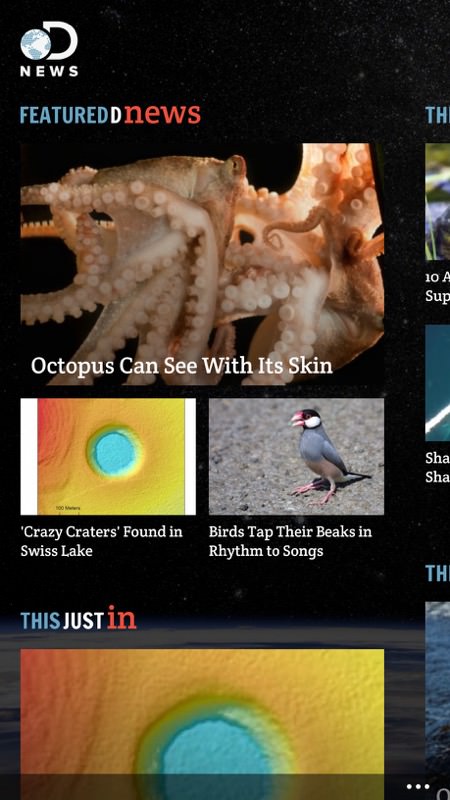This is a detailed caption for an image description:

The image is a screenshot from a phone, presented in a vertically elongated rectangular shape. The background of the screen is predominantly black, resembling the night sky with a few scattered dots, akin to stars. Near the bottom of the screen, there is a narrow band of Earth's image partially obscured by overlapping picture tabs.

In the top left corner of the screen, there is a small globe icon featuring dark blue and light blue hues representing land and water. This globe is encircled by the letter 'D', which continues around to the bottom, accompanied by the word "news" in white font. Directly below this, the word "Featured" appears in blue text. Adjacent to it, the sequence "D news" is presented with the letter 'D' in the same white color and "news" in red. On the right side of this section, the letters "T" and "H" appear in blue.

Running vertically along the right edge of the screenshot are partial images and text. The top visible image is a fragmented picture, followed by the letters "10A" and "SUP." Below this, another partial image appears with the letters "SHA" repeated twice below it. Further down, another partial picture is present with the letters "TH" and more image fragments seen at the bottom right corner, marked by three white dots.

Prominently featured beneath the "Featured" and "D news" text is a close-up image of a light brown octopus against a black background. The caption "octopus" is written in white beneath the image, followed by the phrase "you can see with skin."

Below the octopus image, there are two smaller pictures side by side. The one on the left is bordered in white on both sides, containing a blue circle at the center with yellow above and red to the left. The adjacent image on the right depicts a toucan perched on a concrete surface.

Underneath these images, there are descriptive captions. The left caption reads "Crazy craters found in Swiss Lake" in white text, while the right caption states "Birds tap their beaks in rhythm to songs." Below those, positioned on the left, are the words "this" in blue, "just" in white, and "in" in red. Accompanied by another picture identical to the one described above with a blue circle in the center.